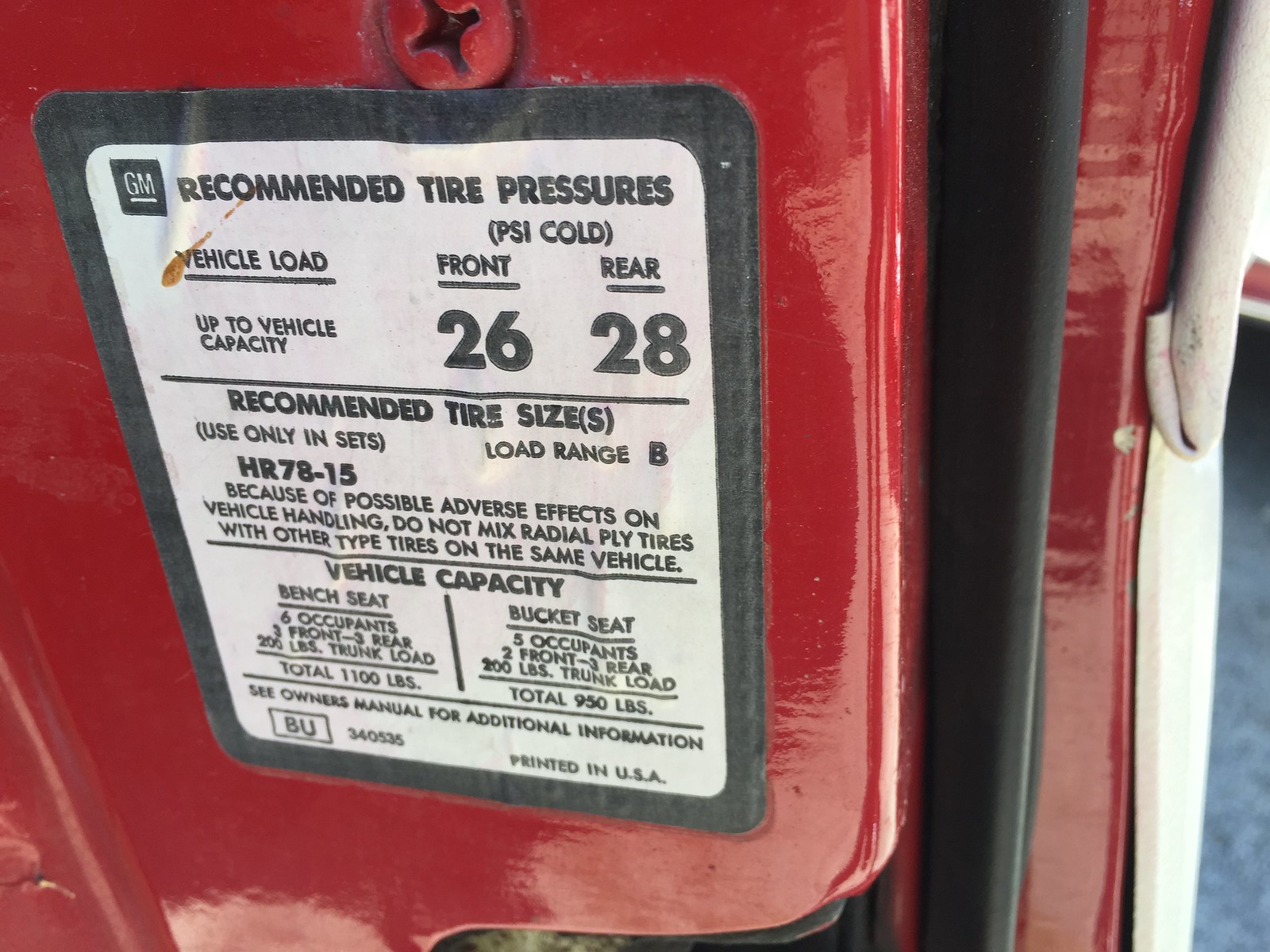This image is a highly detailed, close-up photograph of a sticker affixed to the red metal side panel of a vehicle, possibly an air pump or a gas station fixture. The focal point of the image is a black and white label positioned centrally but slightly towards the left. The label provides critical information regarding GM recommended tire pressures and vehicle load capacities. The label reads: "GM Recommended Tire Pressures, PSI cold. Front 26, Rear 28. Recommended Tire Sizes: Use Only In Sets, Load Range B, HR 78-15. Because of possible adverse effects on vehicle handling, do not mix radial ply tires with other types on the same vehicle. Vehicle Capacity: Bench Seat (6 Occupants: 3 Front, 3 Rear, 200 pounds), Bucket Seat (5 Occupants: 2 Front, 3 Rear, 200 pounds). Trunk Load: Total 1100 pounds (Bench), 950 pounds (Bucket). See owner's manual for additional information. BU340535. Printed in USA." The colors in the image include red, black, white, gray, brown, and green, enhancing the detailed and vibrant presentation of the label and the red metal surface. The photograph appears to have been taken outdoors, focusing on the central label against the vehicle's side panel.